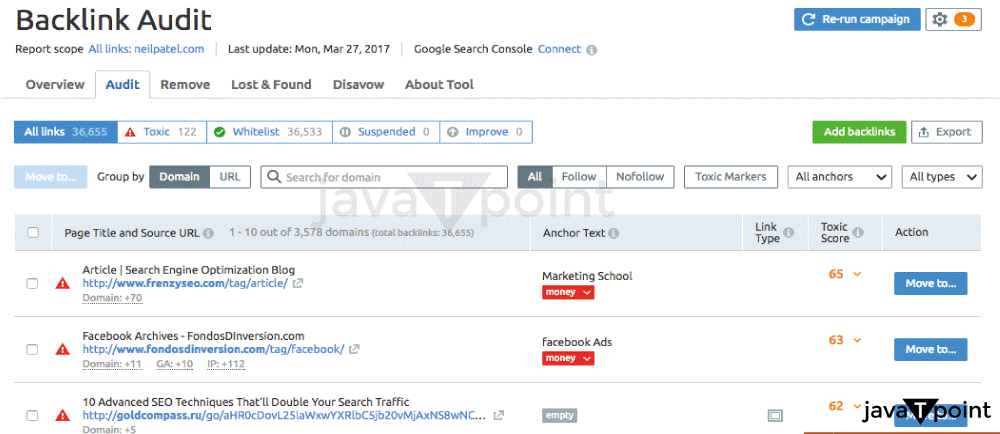### Detailed Caption:

The image is a comprehensive screenshot of a "Backlink Audit" page interface. At the top left corner, prominently displayed, is the title "Backlink Audit," accompanied by a brief explanation that outlines the report scope: "All links neilpatel.com." It also includes a timestamp indicating the last update: "Monday, March 27th, 2017." Just below the scope, there's an option labeled "Google Search Console," offering a link for users to connect their Google accounts.

In the top right corner, two distinct buttons are situated. The first button, "Rerun Campaign," features a blue background with white text and an arrow icon that resembles the redo icon commonly seen in Microsoft Word. Right beside it, there's a white button with a settings cog icon and the number "3" in orange, indicating some configurable options or notifications.

Below these controls is a navigation bar with six options: Overview, Audit, Remove, Loss and Fail, Disavow, and About Tool. The "Audit" option is highlighted in blue, signifying the current page, while the other options are grayed out.

Further down the page, there’s a detailed table for users to inspect various attributes of their backlinks. The table columns include Page Title, Source URL, Anchor Text, Link Type, Toxic Score, and Action, among others. Additionally, users have the functionality to view all links or group the data by domain or URL. Towards the right side of the table, there are two more options for users to either add backlinks or export the data.

This interface provides a thorough and user-friendly platform for managing and auditing backlinks effectively.